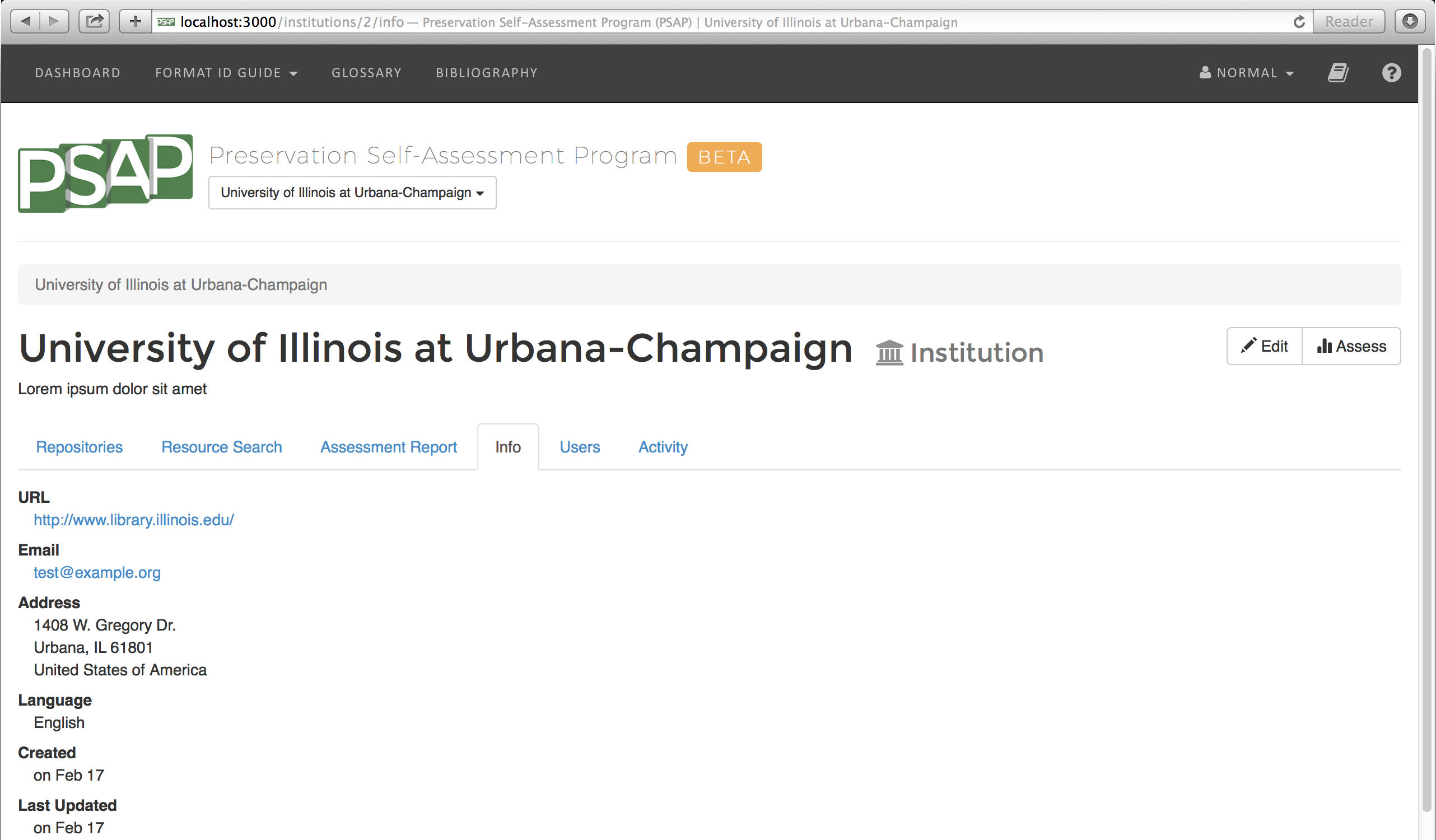This image appears to be a screenshot from a computer displaying information related to a program from the University of Illinois at Urbana-Champaign. In the upper left-hand corner, there is a green shape resembling a waving flag, with the white letters "PSAP" on the green background. "PSAP" stands for Preservation Self-Awareness Program.

Below this emblem, the indicator bar reads "University of Illinois at Urbana-Champaign." Prominently, in larger black letters on a white background, it states "University of Illinois at Urbana-Champaign Institution."

On the left-hand side of the image, additional details are listed, including a URL for the Library of Illinois (library.illinois.edu), an email address, and a physical location: 

1408 West Gregory Drive, 
Urbana, Illinois 61801, 
United States of America.

The language used is English. The creation and last update date are both noted as February 17. All of this information is arranged clearly, predominantly in black lettering on a white background.